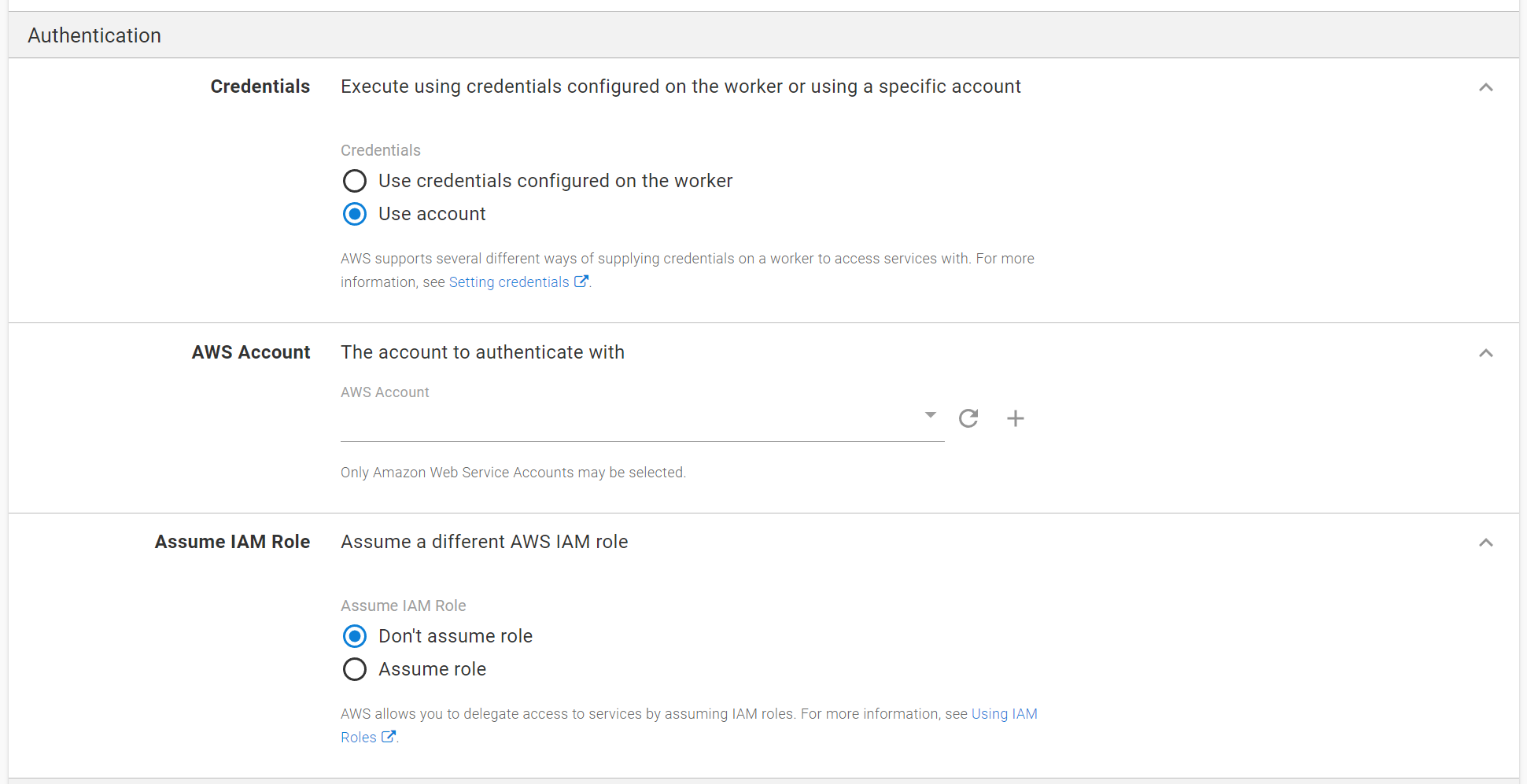A detailed caption for the image of the Authentication Page could be:

---

The image displays an Authentication Page, prominently titled "Authentication" at the top. Below the title, the page is divided into several sections: 

1. **Credentials Section**: This section provides options for executing using credentials. It states, "Execute using credentials configured on the worker or using a specific account." There are two options available:
   - "Use credentials configured on the worker"
   - "Use account" (this option is selected, indicated by a blue-circled button)

   Beneath these options, an informational note explains, "AWS supports several different ways of supplying credentials on a worker to access services with." It also includes a clickable link labeled "settings credentials" for more information.

2. **AWS Account Section**: This section allows selection of the AWS account to authenticate with, featuring a dropdown menu to choose from available accounts. There is a refresh button next to the dropdown box, and a plus sign indicating the option to add accounts. The note below reads, "Only Amazon Web Service accounts may be selected."

3. **Assume IAM Role Section**: In this section, users can choose whether to assume a different AWS IAM role. The available options are:
   - "Don't assume role" (selected, with a blue-circled button)
   - "Assume role"

   An accompanying note explains, "AWS allows you to delegate access to services by assuming IAM roles," and provides a clickable link labeled "using IAM roles" for further information.

---

This detailed description thoroughly covers the layout and functionalities illustrated on the Authentication Page image.